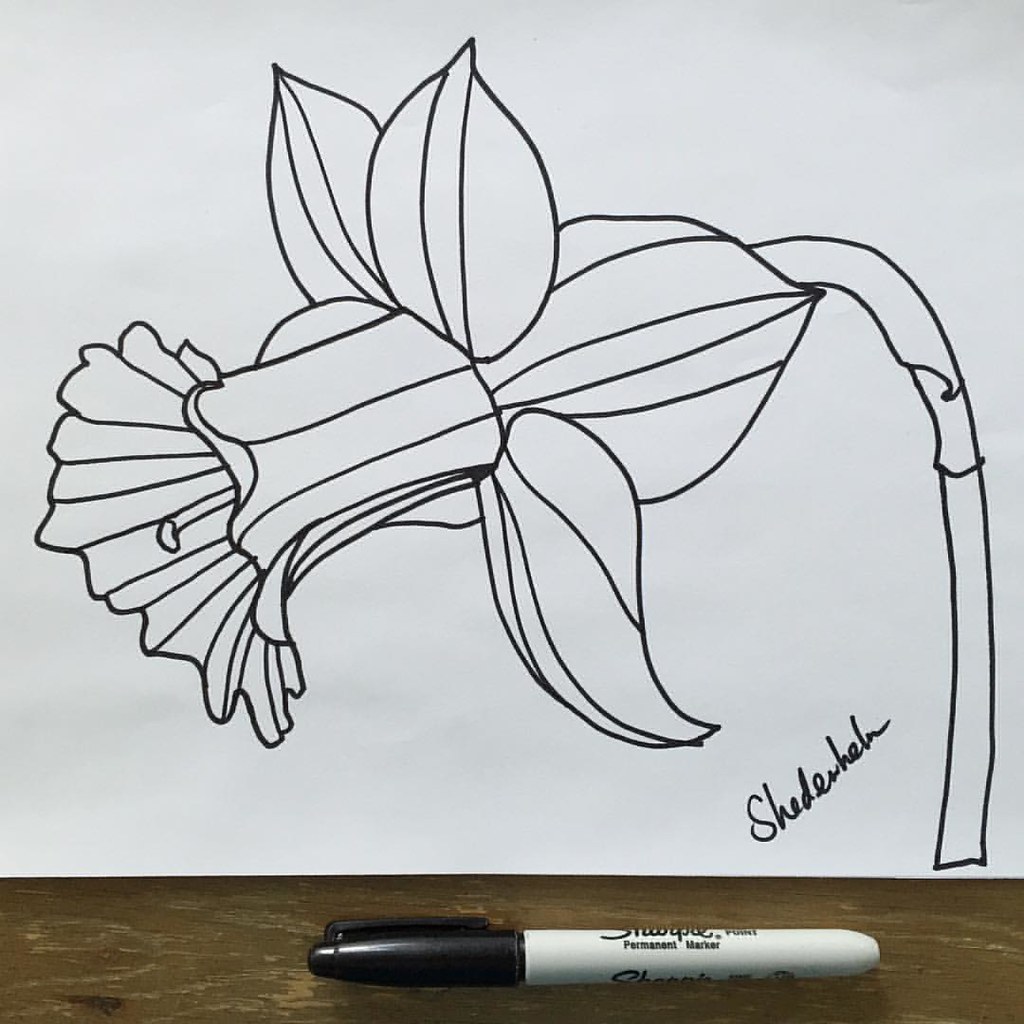On a brownish desk, there is a permanent Sharpie marker placed prominently. Above the marker, a sheet of drawing paper is visible. On the paper, someone has drawn a flower using the Sharpie. The flower is oriented slightly sideways, giving a partial side view. The drawing includes the stem, the bottom petals, and a detailed center. The different areas of the flower are distinct, but the illustration is not shaded; it relies solely on the lines to define its form. The bottom edge of the paper is slightly cut off, revealing more of the desk below.